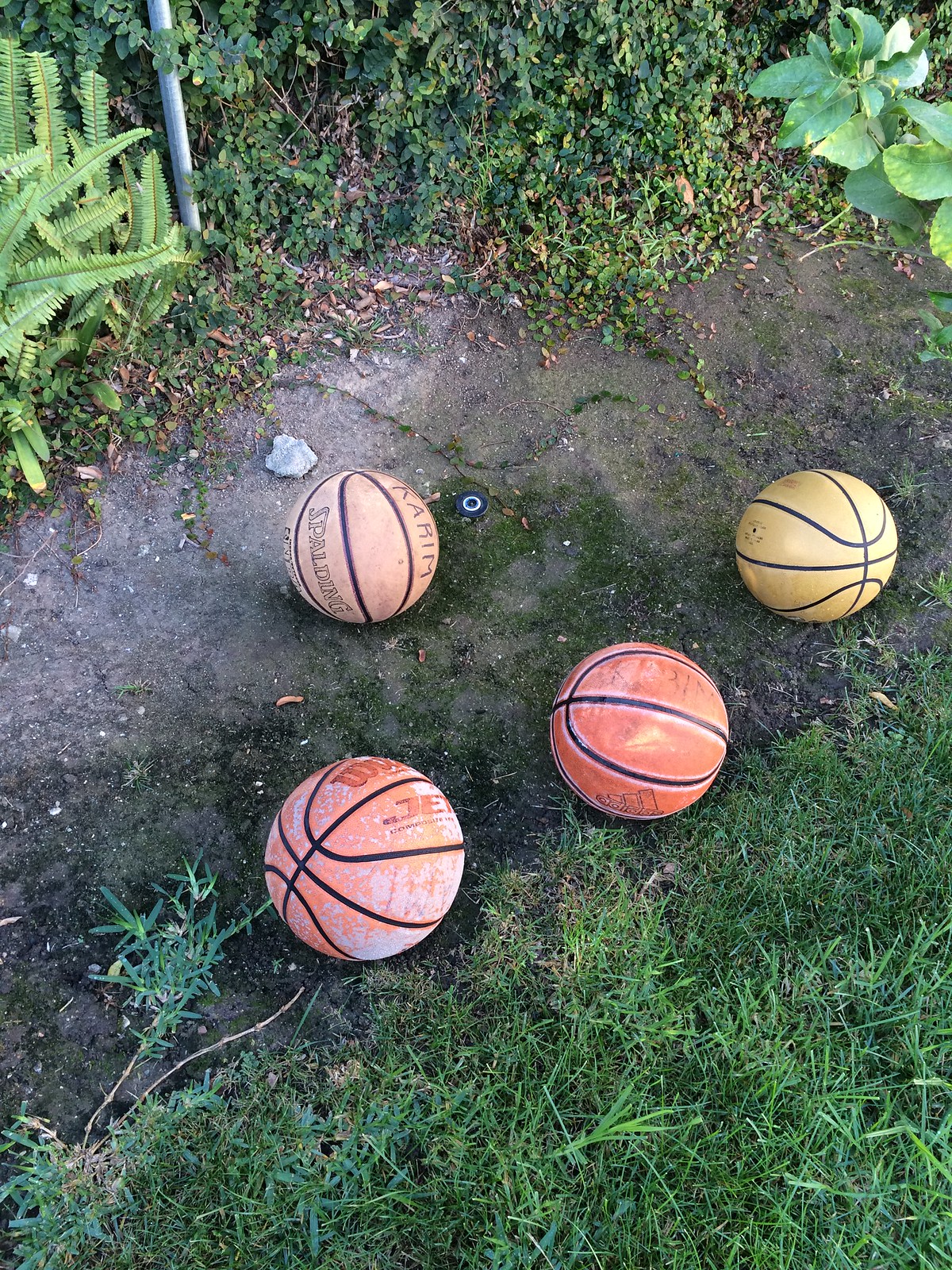This photograph, taken from an overhead perspective, captures four basketballs positioned on a light brown dirt patch with scattered moss. The two basketballs at the bottom exhibit a classic orange hue, while the top two are significantly faded, with one nearing a yellow tint. Visible brand markings identify the balls as Wilson and Spalding, with noticeable wear suggesting extensive use. Surrounding the basketballs is a varied green landscape: on the left, a dense sword fern; to the right, large-leaved plants, and below, a vibrant grassy section. A small black plastic sprinkler head with a white center emerges from the soil near the bottom left basketball. A small rock lies behind the Spalding-labeled basketball, hinting at a casual backyard setting.